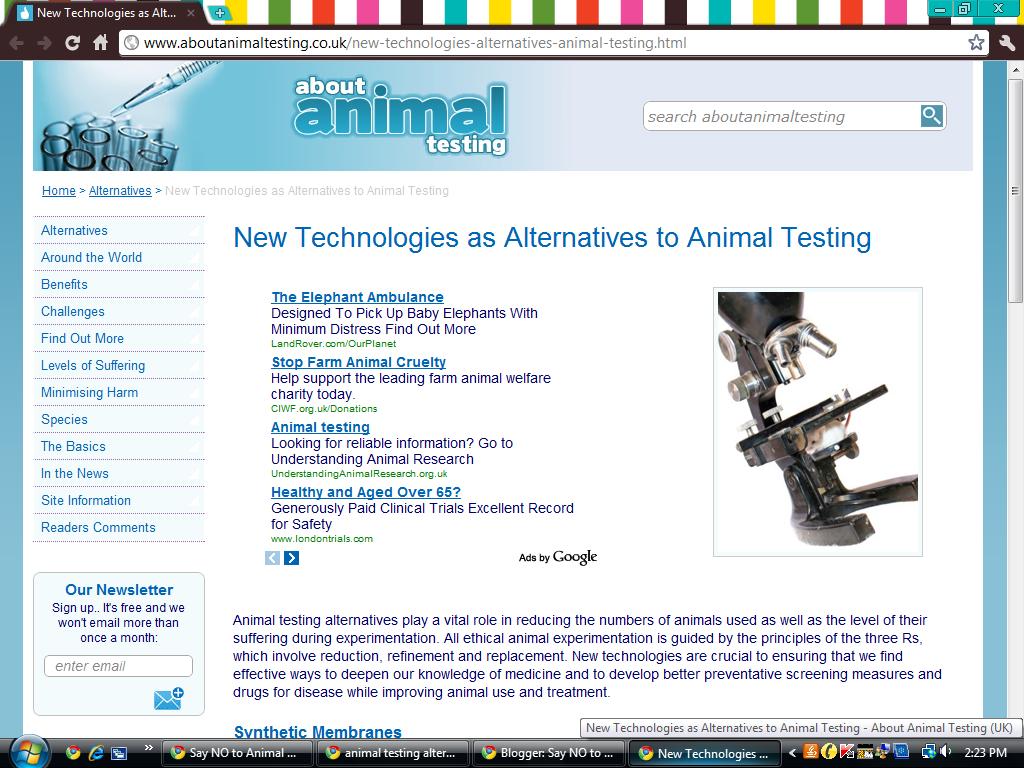The image showcases a website displayed on a browser tab, likely in Chrome or Firefox, indicated by the visible URL section at the top and the Chrome icon on the Windows taskbar at the bottom. The taskbar also displays the time as 2:33, the internet connection icon, and the Windows logo.

The webpage is themed mainly in white and blue hues with navy blue text, focusing on the topic of animal testing. At the top, the header reads "About Animal Testing," accompanied by an image depicting beakers being filled. Adjacent to this, a search box labeled "Search about animal testing" with a magnifying glass icon is visible.

Below the header, the text starts with "New technologies as alternatives to animal testing." Adjacent to this, there are Google ad links and an image of a magnifying glass over a petri dish. The subsequent paragraph elaborates on the importance of alternatives to animal testing, emphasizing their role in minimizing the number of animals used and reducing their suffering. It outlines that ethical animal experimentation adheres to the principles of the three R's: reduction, refinement, and replacement. The text further explains how new technologies are vital for advancing medical knowledge, developing better preventative measures, and improving the treatment and use of animals in research.

On the left side of the page, there is a pane with various sections such as "Alternatives Around the World," "Benefits," "Challenges," "Find Out More," "Levels of Suffering," "Minimizing Harm," "Species," "The Basics," and "New Site Information." Beneath this, a box invites visitors to subscribe to a newsletter.

Overall, the image provides a detailed view of a website dedicated to educating and informing visitors about animal testing and the new technologies that serve as alternatives.